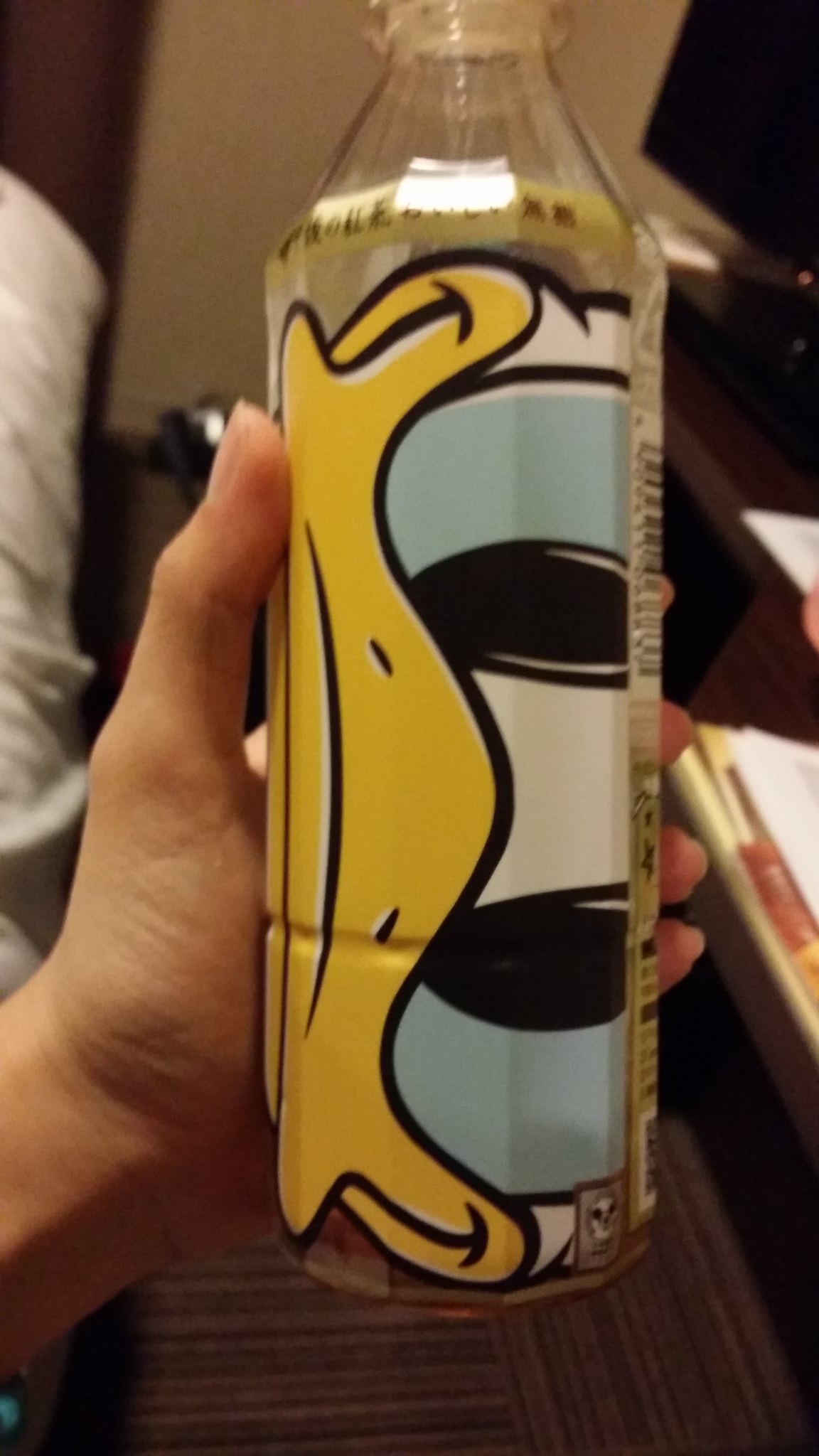Captured in a vertically rectangular frame under dim interior lighting emerging from the lower left corner, this image features a left hand extending upward at an angle. The hand, palm up with the thumb pointing vertically, grasps a slim, tall plastic bottle. The bottle is clear, revealing a partial, sideways depiction of a cartoon duck character. Only the duck's eyes—characterized by blue irises with black pupils—are visible along with the white space between them and its prominent yellow bill. The duck's face appears vertically aligned on the bottle, adding a whimsical touch to the scene.